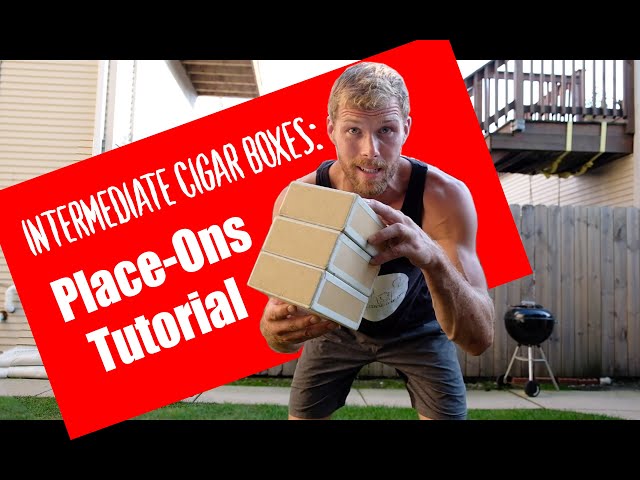In this landscape-oriented, color photograph, a young, muscular man around 25 years old is the focal point, crouching slightly and looking up at the viewer with a half-smile. He has blonde hair, a beard, and a mustache, and he is dressed in a blue tank top featuring a white graphic on the chest and dark gray shorts. The man holds a stack of three small, beige cigar boxes with some white elements, positioned in front of his chest. Behind him is a red horizontal rectangle angled toward the bottom left, overlaying the scene with the white text "Intermediate Cigar Boxes: Place-Ons Tutorial." The detailed backyard setting includes a well-maintained lawn, a yellowish vinyl-sided building with a white gutter, a wooden balcony on the right, a charcoal Weber grill on the sidewalk below it, and an unpainted wooden fence in the background. The image employs photographic realism and graphic design typographic elements.